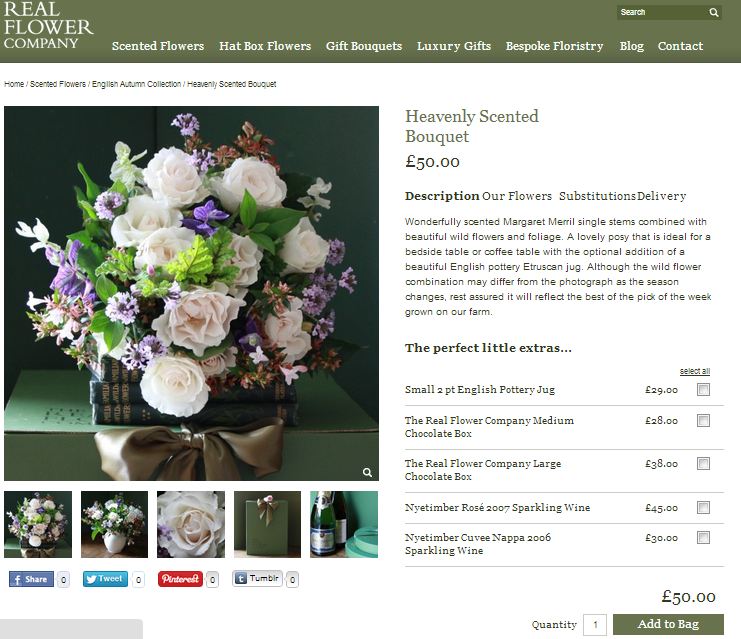The photographic image displays a web page with a header featuring a dark green banner bearing the text "Real Flower Company" in white writing. At the top of the page, there are several categories listed in white text, including "Scented Flowers," "Hat Box Flowers," "Gift Bouquets," "Luxury Gifts," "Bespoke Floristry," "Blog," and "Contact." A search bar with a magnifying glass icon is also present.

On the left side of the page, there is a large photograph showcasing an elegant flower arrangement. The arrangement is placed atop a stack of black, antique-looking books and adorned with a large satin brown bow on the front. The bouquet includes an assortment of flowers such as white roses, white carnations, green ferns, and features some white elongated flowers extending from the top and sides. Additionally, there are small clusters of purple and pink flowers interspersed throughout. The composition also includes loose petals scattered around the arrangement.

Below the photograph, a description reads: "This is a heavenly scented bouquet" with a pricing detail of "50 Euros."